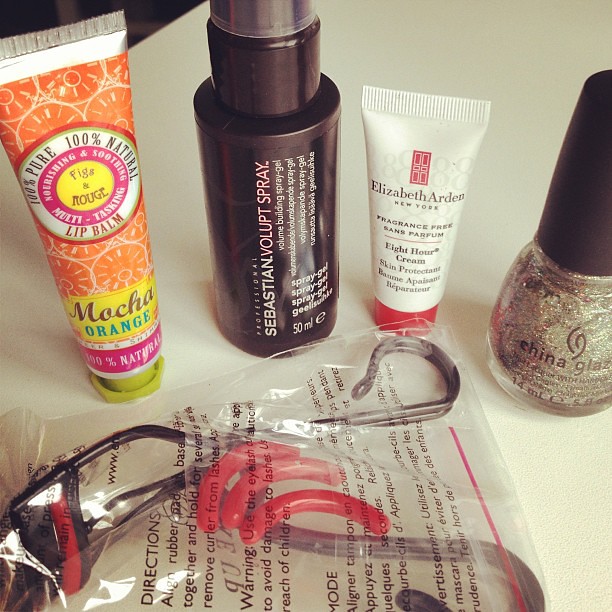The photograph showcases an array of five distinct beauty products meticulously arranged on a pristine white surface with a curved edge, likely part of a counter, desk, or table. Starting from the left, the first item is an orange tube standing upright on its green cap. The tube is emblazoned with various descriptors, prominently featuring "100% natural," "nourishing and soothing," and "multitasking figs and rouge lip balm, mocha orange." Adjacent to it is a brown, plastic bottle with a spritz top capped with a plastic cover. Its label reads "Sebastian Villupt Spray," identified as a "volume building spray gel." Continuing to the right, there is a bottle of "China Glaze" nail polish. Next to this is a container labeled "fragrance-free cream," marketed as a "skin-protecting cream." The final item is a small plastic bag which contains an eyelash curler along with rubber pads and specific usage directions detailing how to line the rubber pads and hold for several seconds before removing the curler from lashes. The overall composition clearly emphasizes a varied selection of beauty and cosmetic essentials.